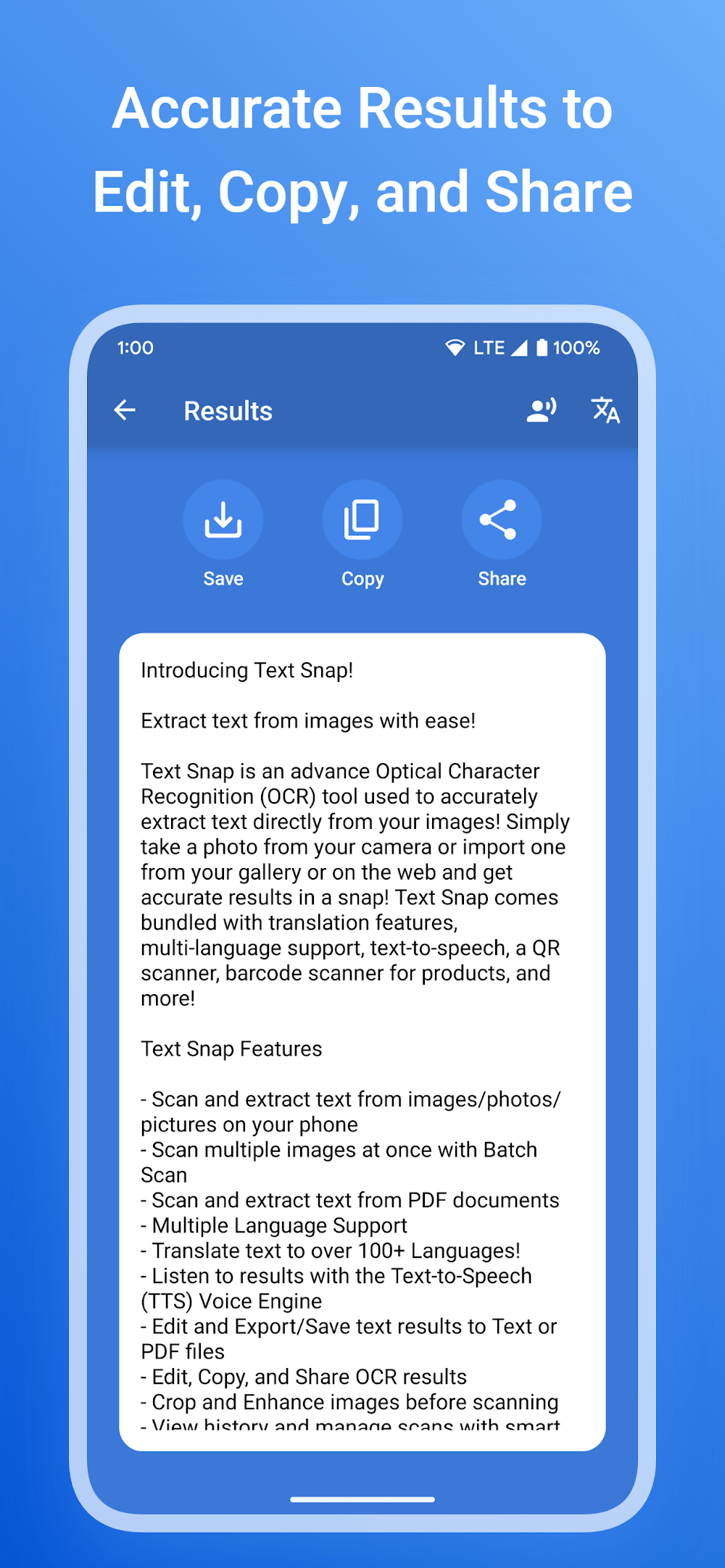The image features a predominantly blue screen designed in the shape of a vertical rectangle. The background of the screen is blue, with prominently displayed white text stating, "Accurate results to edit, copy, and share." 

Central to the image is a framed imitation of a smartphone screen, bordered in a light blue frame. At the top of this screen, the time is shown as 1:00, and various icons indicate a mostly filled Wi-Fi signal, full LTE signal strength, and a 100% battery level. 

Beneath these indicators is a navigation bar, which includes the word "Results" accompanied by a leftward arrow, followed by an icon of a person with audio waves (indicating text-to-speech), and the Google Translate icon further right.

Below the navigation bar, three buttons are visually lined up: a save button, a copy button, and a share button, each with their respective icons. 

Further down in the main content area, there's a white text box that reads:

"Introducing TextSnap. Extract text from images with ease. TextSnap is an advanced optical character recognition (OCR) tool used to accurately extract text directly from your images. Simply take a photo from your camera or import one from your gallery or the web to get accurate results in a snap. TextSnap comes bundled with translation features, multi-language support, text-to-speech, a QR scanner, barcode scanner for products, and more. 

TextSnap features: 
- Scan and extract text from images/photos/pictures on your phone.
- Scan multiple images at once with batch scan.
- Scan and extract text from PDF documents.
- Multiple language support.
- Translate text to over 100+ languages.
- Listen to results with the text-to-speech (TTS) voice engine.
- Edit and export/save text results to text or PDF files.
- Edit, copy, and share OCR results.
- Crop and enhance images before scanning."

The description cuts off at this point, and the image concludes with no further information shown.